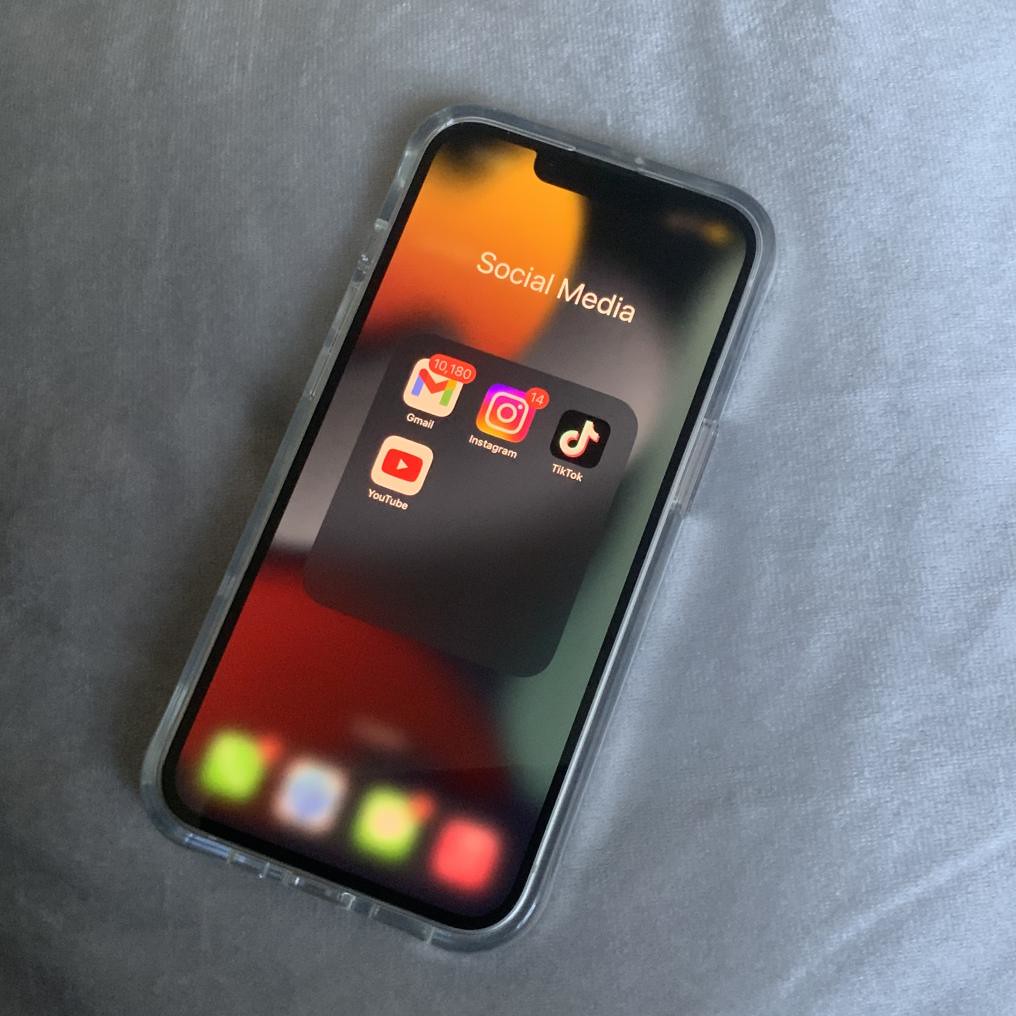This photograph showcases an iPhone resting on a blue cloth backdrop. The device, encased in a clear plastic protective case, prominently displays its social media folder open on the screen. Within this folder, there are four visible apps: YouTube, Gmail, Instagram, and TikTok. The surrounding icons and screen elements are blurred, drawing focus to the social media applications. The iPhone model appears to be an iPhone 8 or later, based on its design and structure, though the exact model remains uncertain.